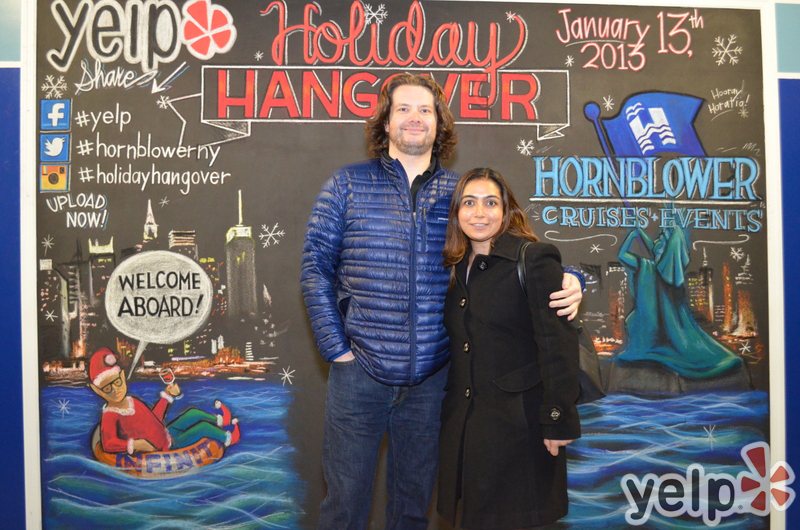In this image, a man and woman are posed against a detailed mural in a festive, urban backdrop. The man, a white male with long, shoulder-length red hair and a scruffy beard, is dressed in a royal blue puffer jacket and blue jeans. He stands with his arm around the woman, who is wearing a black wool coat with buttons and has long brown hair, just reaching his shoulder. The mural behind them features an elf floating in an orange and white striped inner tube, holding a glass of wine. Above the elf is a speech bubble that says "Welcome Aboard." 

The mural is peppered with various social media logos and hashtags: Yelp, Facebook, Twitter (#HornblowerNewYork), Instagram, and Snapchat (#HolidayHangover), along with the directive "Upload Now." In red, bold letters, the mural reads "Holiday Hangover," with an accompanying date, January 13, 2013, in light pink in the upper right-hand corner. Beneath the headline, it mentions "Hornblower Cruise Events" and "Yelp" symbolically on both sides. The Statue of Liberty is also depicted holding a flag with an 'H' on it, set against a cityscape background adorned with snowflakes. The water in the mural is rendered in blue, contrasting the primarily black city skyline.